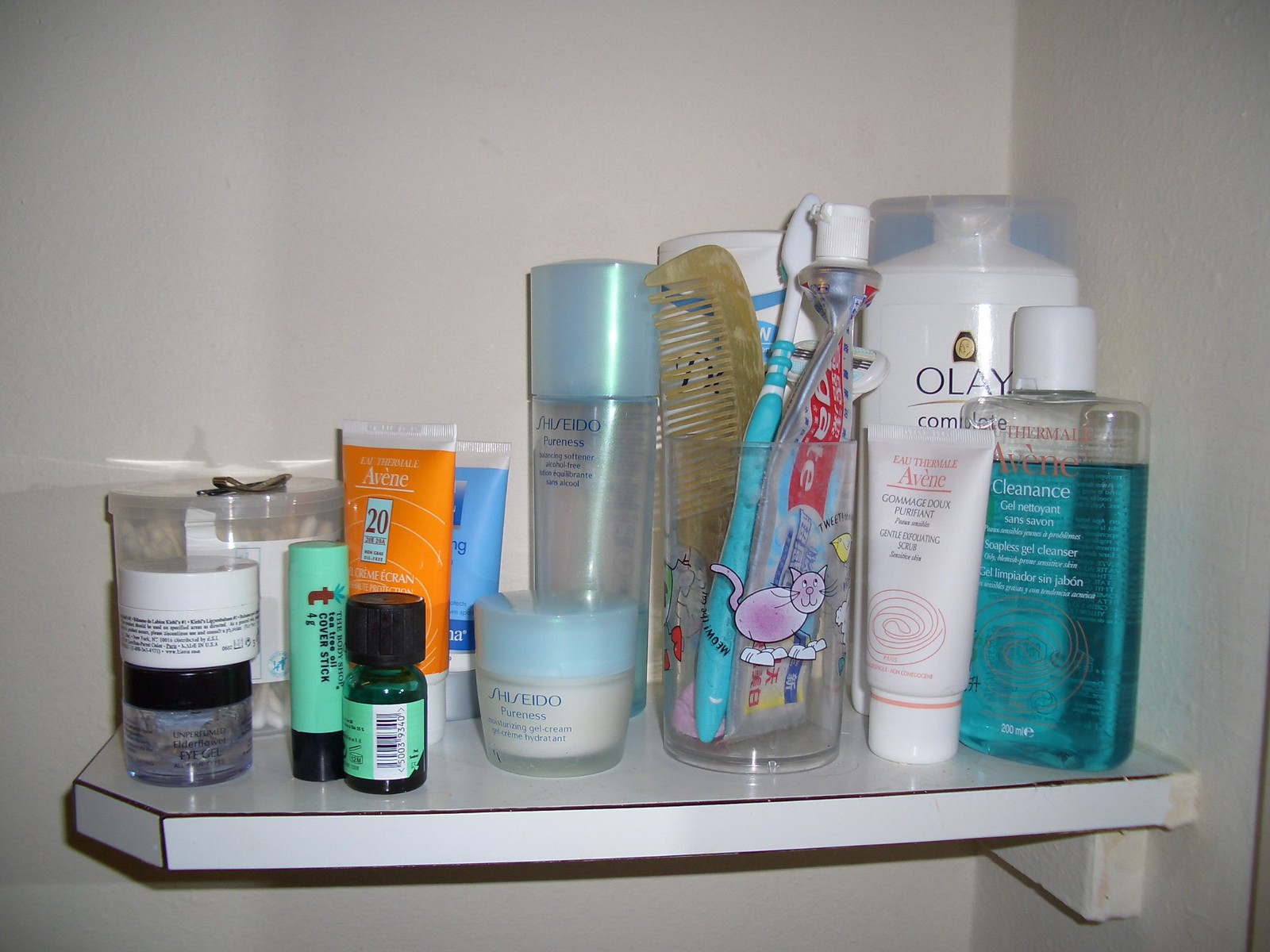The image depicts a white bathroom shelf, meticulously organized with an array of personal care items. Starting from the right side, there is a clear gel with a blue label. Moving towards the center, one can spot a white bottle containing lotion cream, distinctive with its label. Adjacent to it is a small white bottle, possibly a travel-sized product. 

A glass cup near the middle of the shelf holds several toothbrushes and a tube of toothpaste, along with a needle brush towards the back left. Below, a product with a blue cap, possibly cream, takes its place on the bottom left. 

Also on the left, sits a mini bottle with a black cap and a green body, next to which is an orange lotion container. To complete the spectrum of colors, a blue lotion bottle is seen, accompanied by a light green, mint-flavored lip gloss or similar product. The shelf's backdrop is a pristine white, highlighting the variety of items neatly arranged upon it.